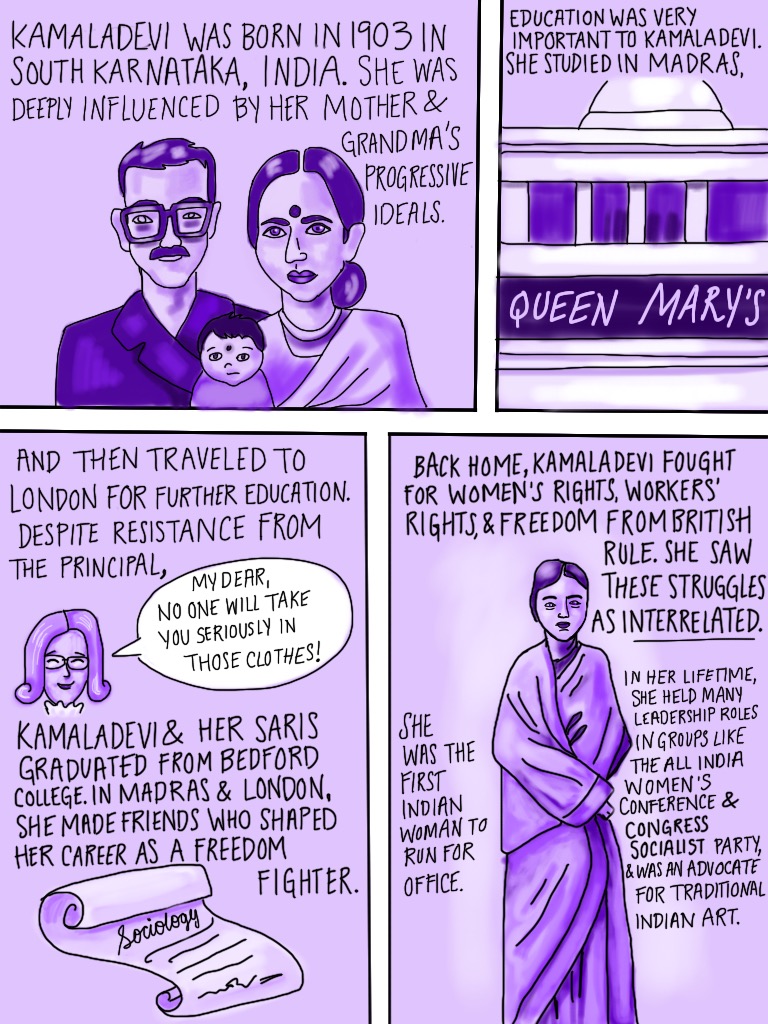This illustration resembles a comic book and chronicles the life of the freedom fighter Kamala Devi. 

In the upper-left corner, there's a depiction of a man and a woman holding a baby, accompanied by the text, "Kamala Devi was born in 1903 in South Karnataka, India. She was deeply influenced by her mother and grandmother's progressive ideals."

To the right, an image of a white building is shown with the caption, "Education was very important to Kamala Devi. She studied in Madras at Queen Mary's College."

On the bottom-left, another panel reveals, "She then traveled to London for further education," featuring a woman with a speech bubble stating, "My dear, no one will take you seriously in those clothes." Below this, it reads, "Despite resistance from the principal, Kamala Devi, in her traditional sari, graduated from Bedford College."

Further to the right, Kamala Devi is depicted standing in her sari. The accompanying text reads, "Back home, Kamala Devi fought for women's rights, workers' rights, and freedom from British rule, viewing these struggles as interrelated. She was the first Indian woman to run for office, holding leadership roles in the All India Women's Conference and Congress Socialist Party, and advocating for traditional Indian art." 

A scroll labeled "Sociology" and a depiction of Kamala Devi add further context to her achievements and values. 

Each panel within the illustration is adorned with purple coloring, adding a cohesive visual theme to the entire piece.